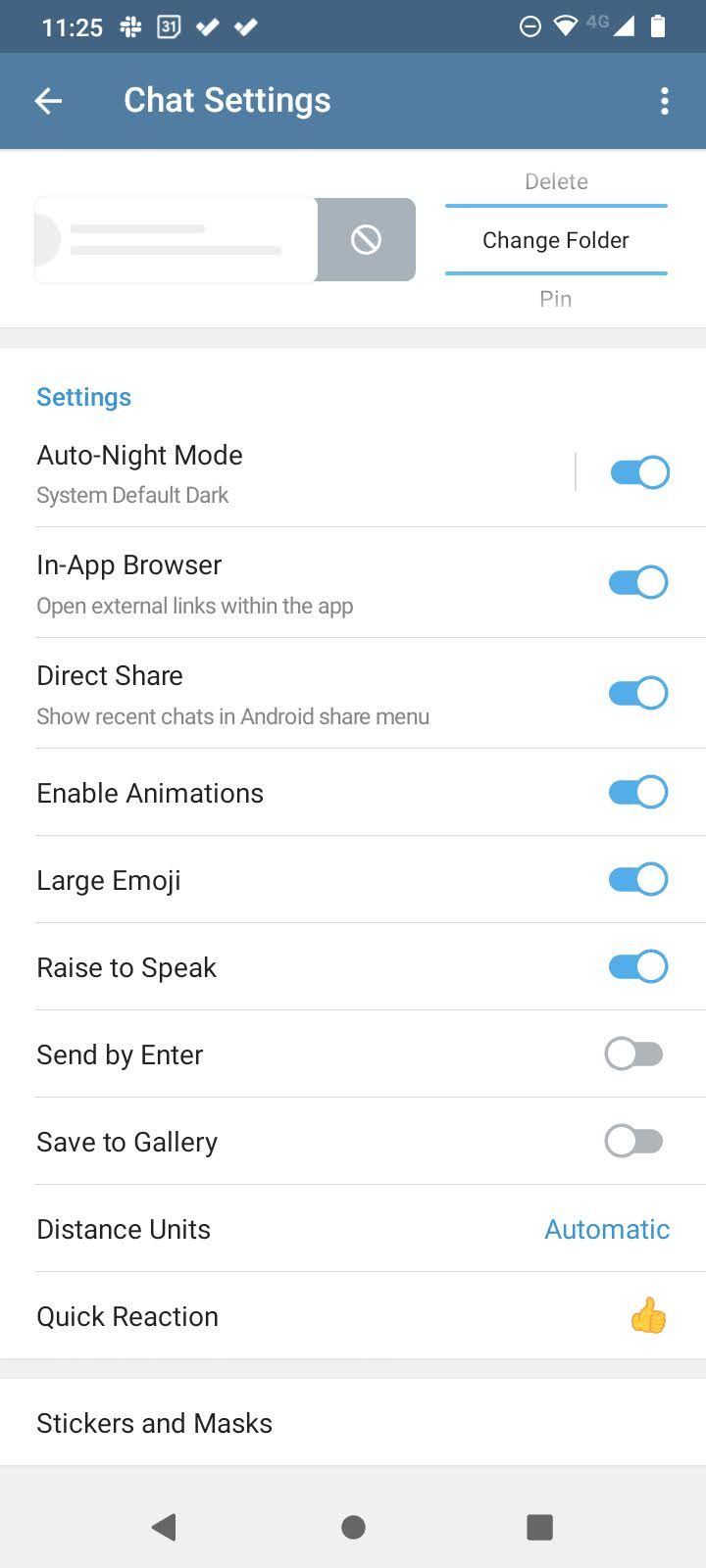The image depicts a smartphone screen with the time displayed at the top, showing 11:25. Adjacent to the time is a unique logo resembling an intricate plus sign, which the user is unfamiliar with. The date '31' and two check marks are also visible. Standard phone icons, such as the Wi-Fi strength bar, 4G indicator, and battery status, are present at the top.

Beneath these indicators, the screen is primarily blue, labeled "Chat Settings." This section provides various configuration options depicted with on/off switches:

1. **Auto Night Mode** - Switch is blue, indicating it is on.
2. **In-App Browser** - Switch is blue, indicating it is on.
3. **Direct Share** - Switch is blue, indicating it is on.
4. **Enable Animations** - Switch is blue, indicating it is on.
5. **Large Emoji** - Switch is blue, indicating it is on.
6. **Raise to Speak** - Switch is blue, indicating it is on.

Following these are settings with gray switches, suggesting they are off:

1. **Send by Enter** - Switch is gray, indicating it is off.
2. **Save to Gallery** - Switch is gray, indicating it is off.

Additional settings include:

- **Distance Units**, which reads "Automatic" on the right.
- **Quick Reaction**, which features a yellow emoji icon next to it. 

Finally, there are options for **Stickers and Masks**, though nothing is displayed to the right of this setting. The screen concludes with typical phone navigation icons: a bar, a circle, and a square, positioned at the bottom.